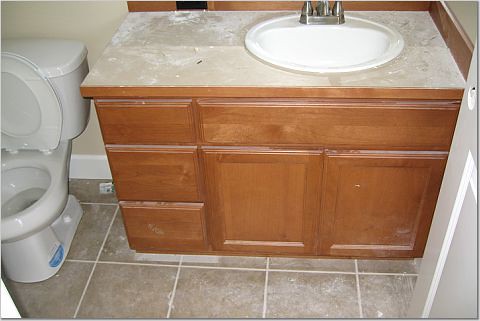This photo captures a bathroom vanity area mid-renovation. The vanity features an oval, inset sink with the faucet and a portion of the backsplash cut off from the frame. The countertop is noticeably dirty with a layer of powder and dust, indicative of ongoing construction work. The vanity itself is crafted from brownish wood and stands out against the taupe-colored walls. 

To the left of the vanity sits a toilet with the seat raised. A noticeable sticker is affixed to the bottom right side of the toilet bowl. The brown tile flooring complements the earthy tones of the room. Adding to the construction atmosphere, an open door without a doorknob is visible, and the general presence of dust underscores the incomplete state of the renovation.